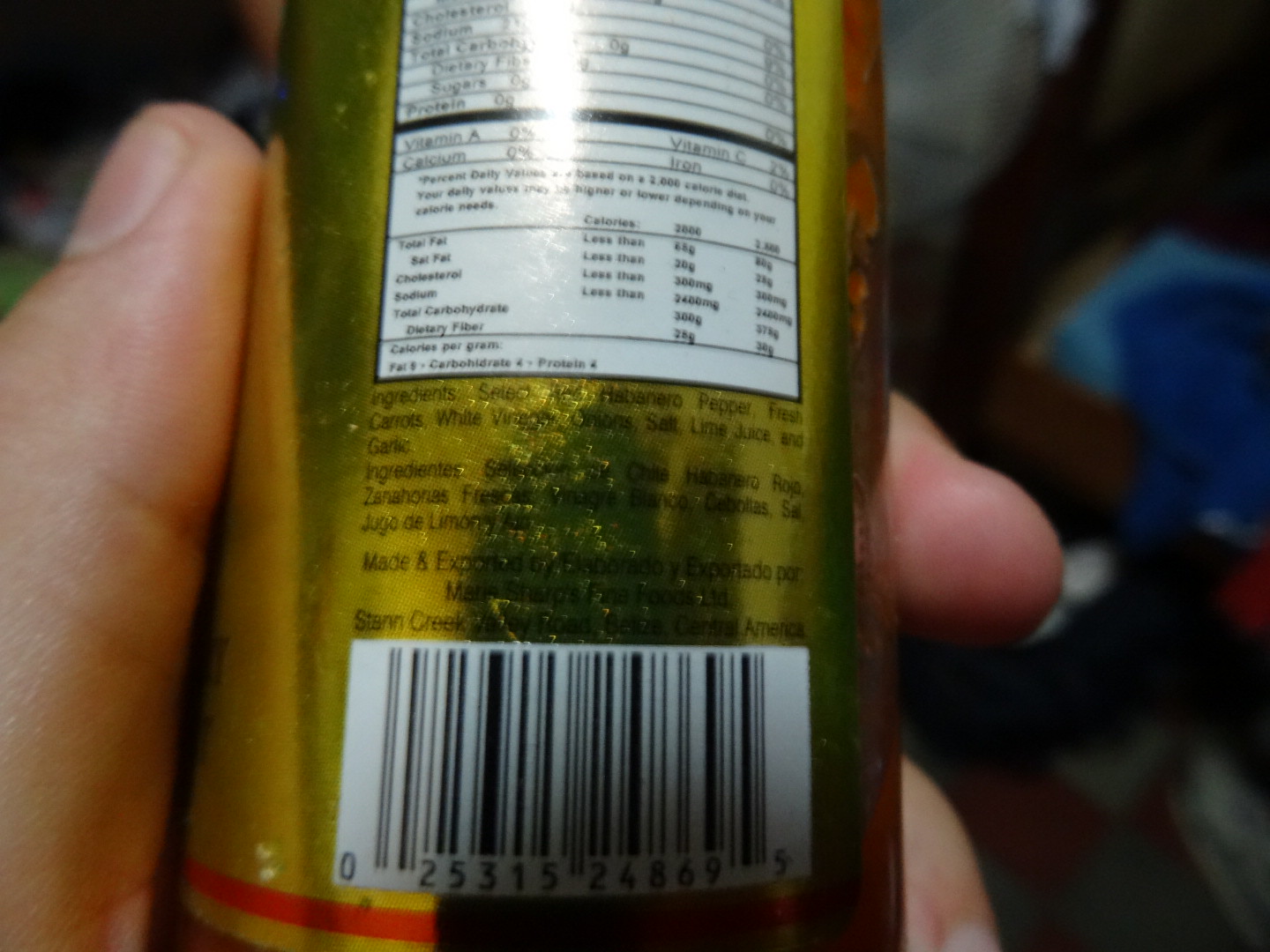The image depicts a person's left hand holding a gold can, resembling a Pringles-type cardboard cylinder. The hand obscures some of the can, with the thumb positioned to the right and fingers wrapping to the left. The can features a red border along the bottom and a red design partially visible on the right side. The background is blurred, yet a blue box is discernible. The can's Nutrition Facts are cut off at the top, starting with the cholesterol line, and are somewhat obscured by glare. What can be read includes Cholesterol less than 300 milligrams, Sodium less than 2,400 milligrams, Total Carbohydrates 300 grams, Dietary Fiber 28 grams, Vitamin A 0%, Vitamin C 2%, Calcium 0%, and Iron 0%. The ingredients listed are Habanero Pepper, Fresh Carrots, White Vinegar, Onion Salt, Lime Juice, and Garlic, with these also repeated in another language. Additionally, there's a barcode at the bottom of the can.